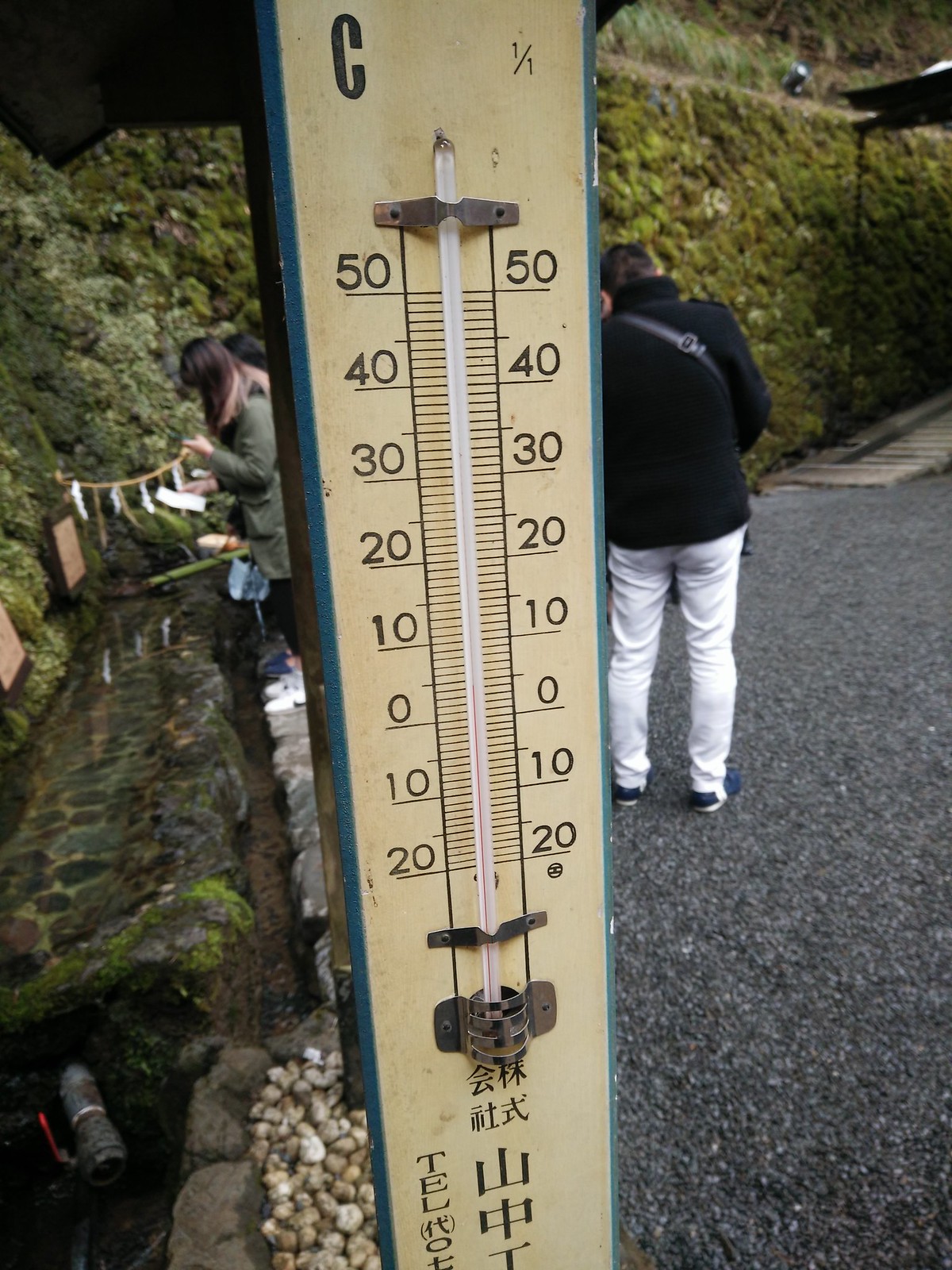In the foreground of the image, a woman wearing a green shirt holds a string with various objects attached to it in one hand and a piece of paper in the other. She is carrying a bag over her shoulder. Rocks are scattered near the bottom of the scene, along with a rusty-looking container that has a red handle. Prominently displayed is a large thermometer with a black side and blue outline, featuring a yellowish interior and a large black letter 'C' at the top. Numbers and lines mark the temperature on the thermometer. 

In the background, there are moss-covered rocks or hedges. On the upper left-hand corner, the scene transitions into darkness. On the upper right-hand side, another person is visible from the back. They are wearing a black jacket, white pants, blue shoes, and have a black purse slung over their shoulder. The setting has a somewhat rustic and natural ambiance, enhanced by the earthy tones and aged materials present.